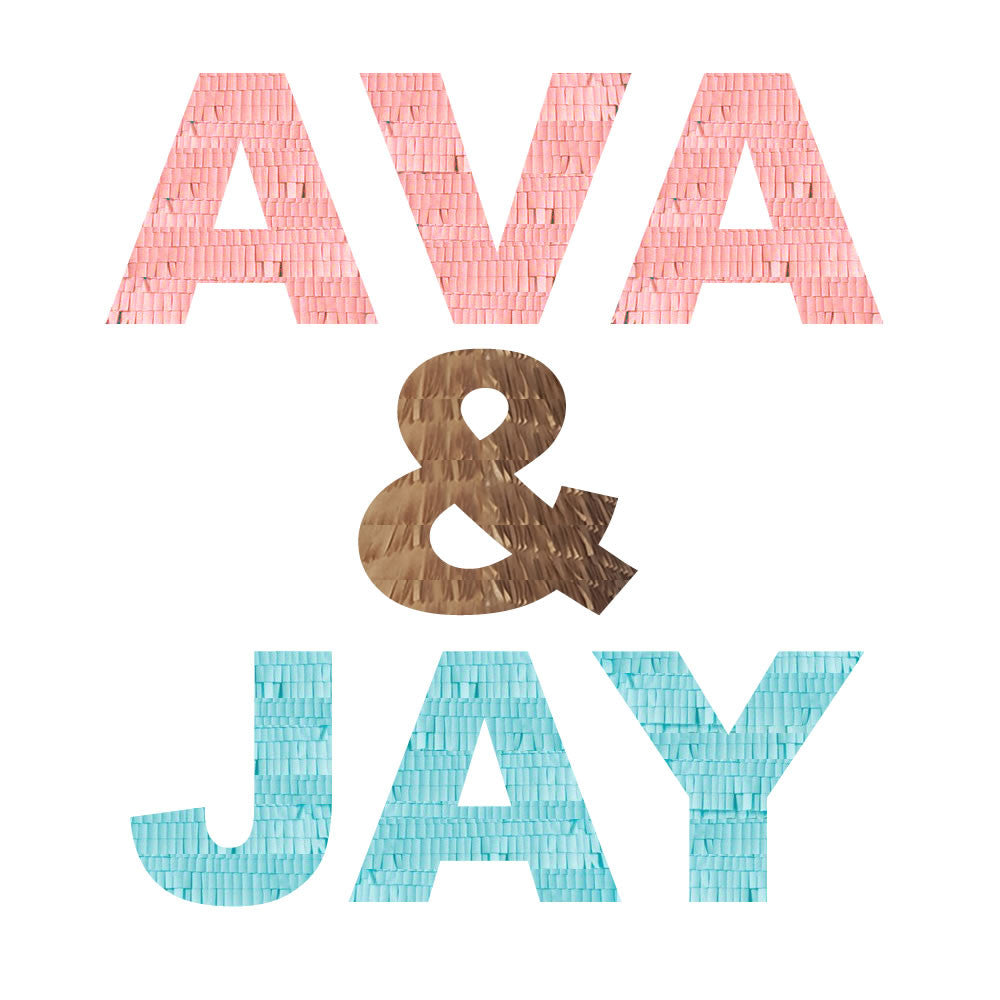The image displays a sign with the names "Ava" and "Jay" in large, capital block letters against a plain white background. "Ava" is written at the top in a rosy pink color and features a textured design resembling small, brick-shaped pieces or shingles. Below it, the word "Jay" appears in a bright sky-blue hue with the same intricate texture. Between the two names, a brown ampersand symbol "&" is present, displaying a slightly different, more stringy or lined texture. The entire arrangement, which looks like it could be a photograph of an actual sign, suggests it might be intended for an engagement party or some celebratory occasion.